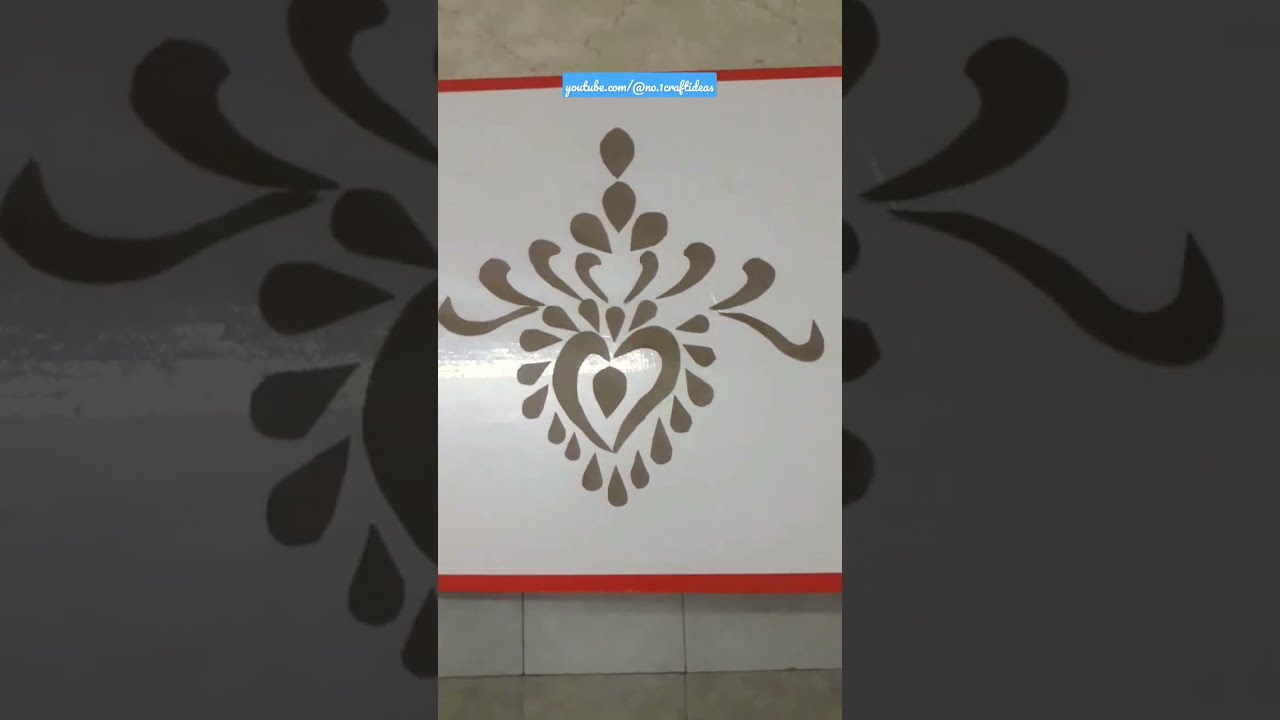The image depicts a detailed painting on a shiny white and grey-tiled wall, bordered at the top and bottom by narrow red-orange stripes. The central piece, a hand-drawn depiction, consists of a grey heart adorned with a diamond-like shape in the center. Surrounding the heart are teardrop motifs and petal-like curves, with larger wave-like petals soaring upwards, giving the impression of a crown. There is a blue rectangle containing white cursive text, "youtube.com/at no.one craft ideas," situated within the upper red-striped border. This central artwork is flanked by enlarged, darkened portions of the same image on its left and right sides, creating a cohesive yet magnified background design. The bottom section of the wall transitions into grey-tiled flooring, adding depth to the scene.